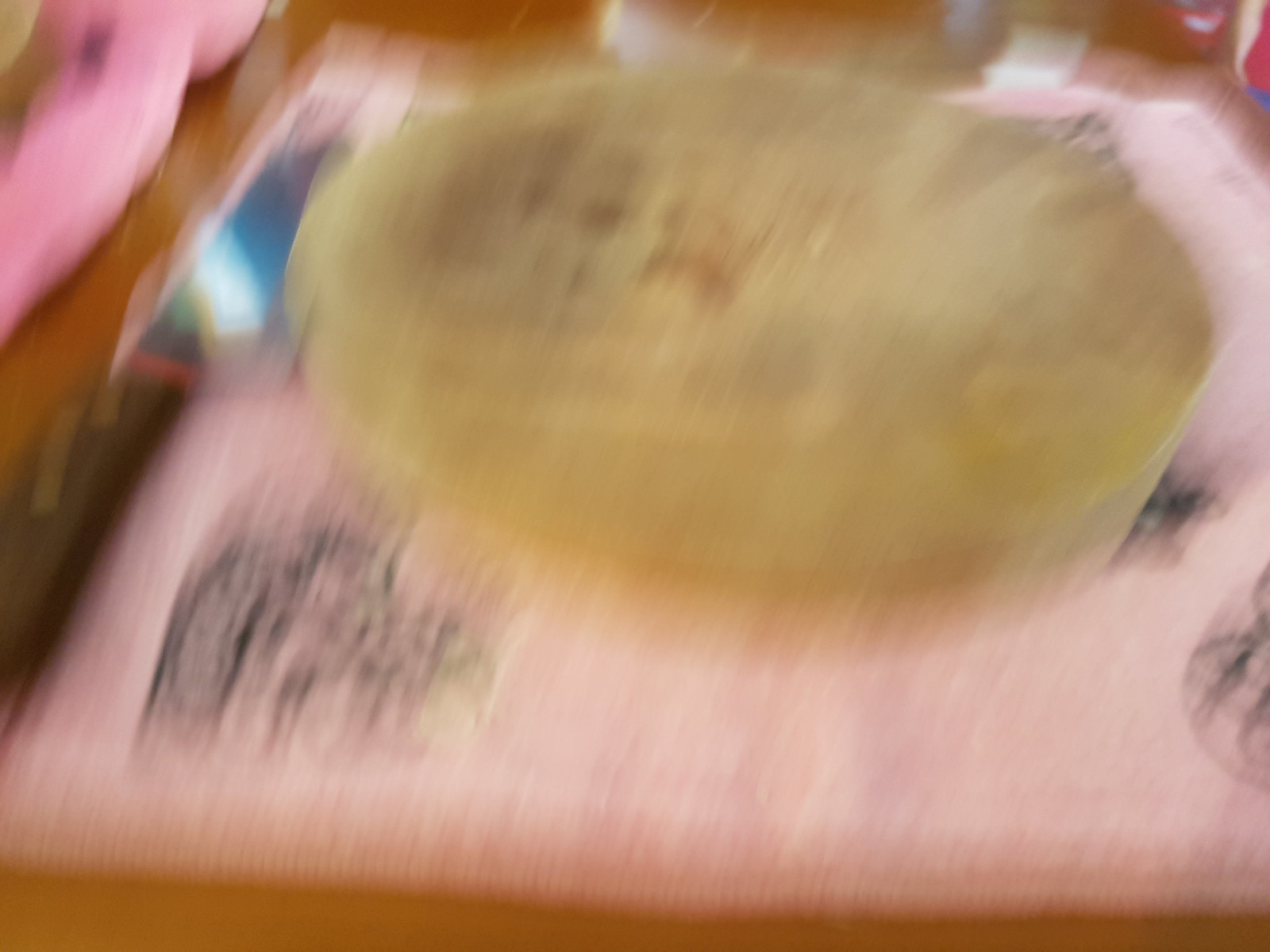This blurry photograph seems to capture an indoor scene with a light-colored hardwood floor. Placed on the floor is a pink mat, which may have a fuzzy texture and possibly sewn edges, reminiscent of a placemat or a small rug. This pink mat appears to have some kind of black design or border. On the left side of the mat, you can spot a knife with a wooden handle and a shiny blade. The centerpiece of the image is a round, yellowish-brown object located on the mat, which lacks clarity but could be anything from a cake to a pillow. The image's extreme blurriness makes it difficult to precisely identify the items and their textures.